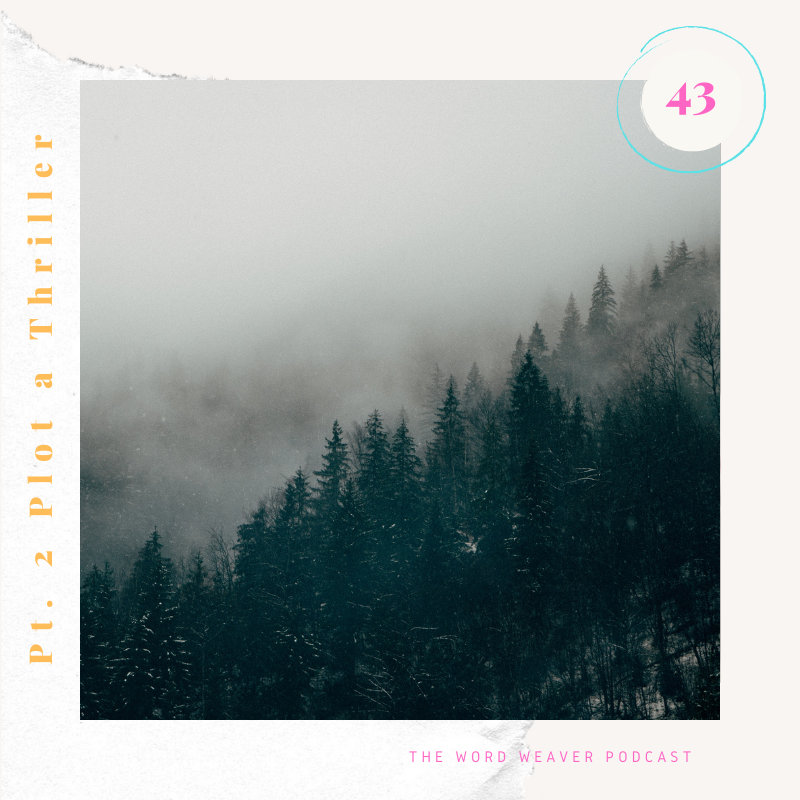This image depicts a foggy, pine-covered hillside and appears to be the cover for a podcast. The entire picture exudes an eerie, dark forest vibe, as it is shrouded in mist, creating an air of mystery reminiscent of an old murder mystery. The main colors in the forest scene are dark green, with hints of snow dusting the trees and ground. The border surrounding the image is white, contributing to a stark contrast with the dark forest.

In the top right corner, there is a circle with a pink number 43 inside, outlined by a turquoise border. This likely signifies the episode number. On the left side, a vertical line of orange text reads “Part Two: Plot A Thriller,” adding to the suspenseful feel of the cover. In the bottom right corner, "WordWeaver Podcast" is written in pink, indicating the title of the podcast. The design elements and coloration enhance the sense of mystery and intrigue conveyed by the fog-laden forest.